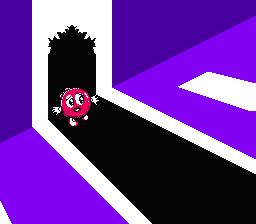This vibrant and playful illustration, reminiscent of a cartoon or video game, depicts a vividly colored scene. On the left side of the image, a wall casts a purple reflection onto the floor, forming a vertical stripe that stretches from the wall to the floor. Adjacent to this, a white stripe extends downward in a similar fashion. To the right, another purple stripe mirrors the one on the left.

In the center of the white stripe lies a jagged, black hole, appearing as if it has been punched through the wall. The darkness pours onto the white floor, contrasting sharply with its pristine surroundings. 

The focal point of the image is a small, purple, round character situated within the black void. This animated figure has expressive eyes and a mouth, with two tiny hands protruding from the sides of its head and two feet extending from its bottom.

Additionally, a white rectangle accentuates the purple floor area on the right side of the composition, adding an extra element of intrigue to the scene.